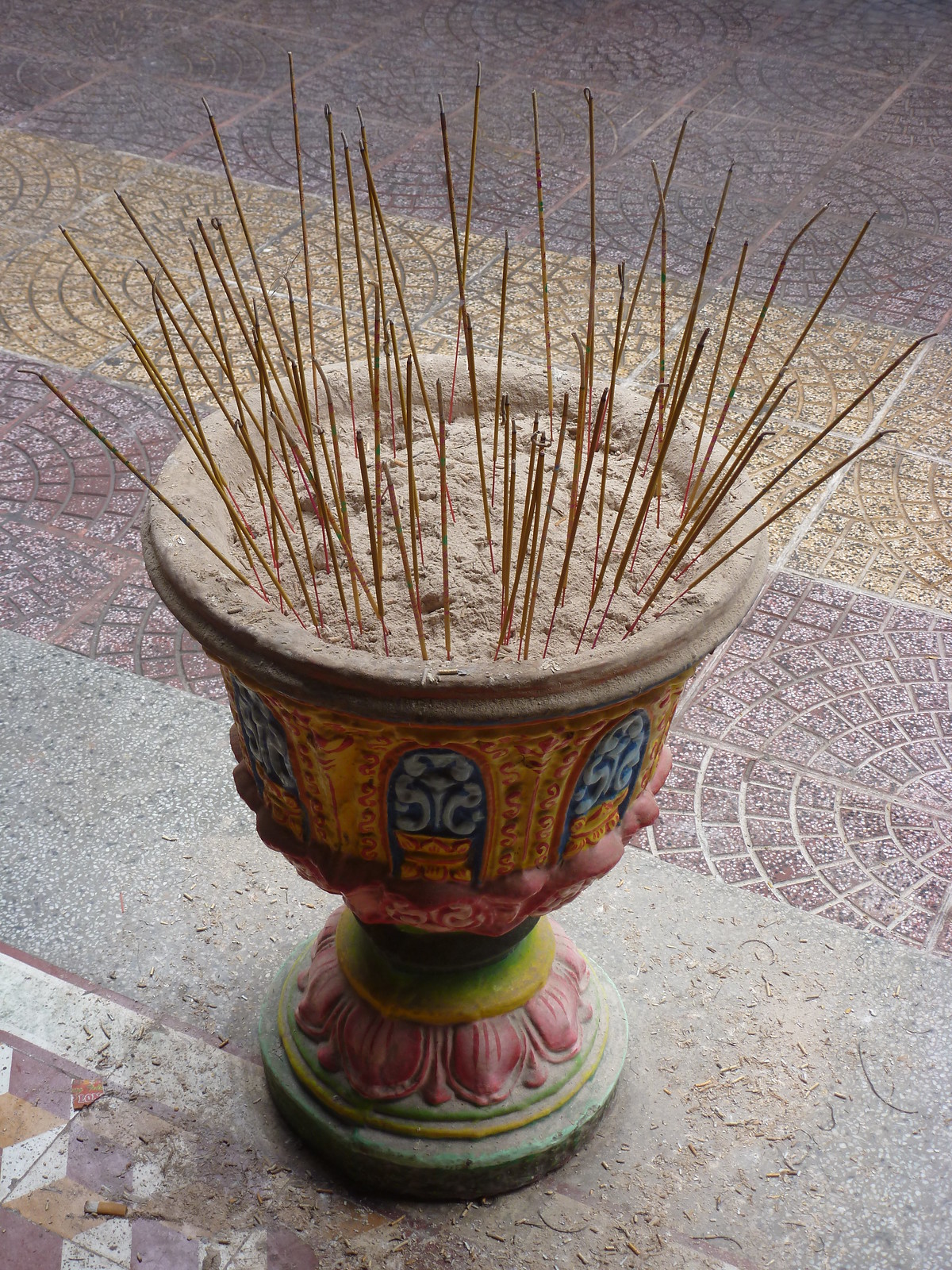This color photograph captures a detailed and vividly decorated urn-style planter prominently positioned on a pastel-colored, mosaic stone walkway. The walkway features a series of concentric circles segmented into squares with subtle hues of golden, purple, gray, and brown. In the foreground, the urn-shaped planter stands out with its elaborate design, characterized by slender, bell-like contours. The planter showcases an ornate relief in a spectrum of colors, including pink, yellow, green, dark blue, sky blue, and orange. At its base, green accents with a pink petal design complement the blue arches and surrounding orange detailing of the body. The urn is filled with sand, slightly mounded at the center, and densely populated with numerous incense sticks, some bearing traces of ash at the ends. This composition of vibrant motifs against the mosaic patio creates an intricate and aesthetically pleasing scene.